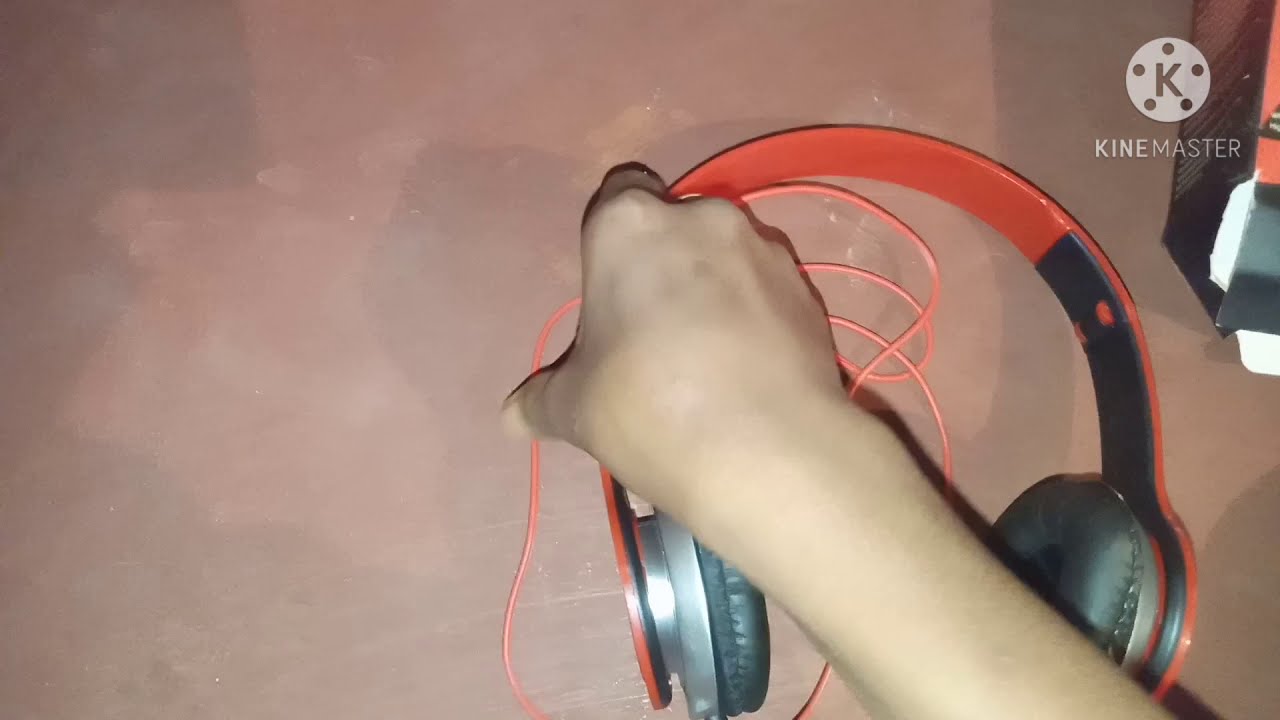The image is a horizontally oriented photograph depicting a light tan-skinned hand coming from the bottom right corner towards the center, grasping a pair of orange and gray headphones. Positioned on a somewhat reddish beige surface with darker shadows, the headphones lie with their earbuds at the bottom and the bands towards the right side of the image. In the upper right corner, an opened gray and orange box – presumably the packaging for the headphones – is partially visible. Above the box, a white circular logo with a K surrounded by five dots can be seen. Directly underneath the logo, in white capital letters, it reads "KINEMASTER." Multiple colors, including orange, gray, silver, tan, purplish-pinkish-brown, white, and reddish-orange, are present throughout the image. Shadows, including that of the person's arm, extend across the surface, suggesting indoor lighting.